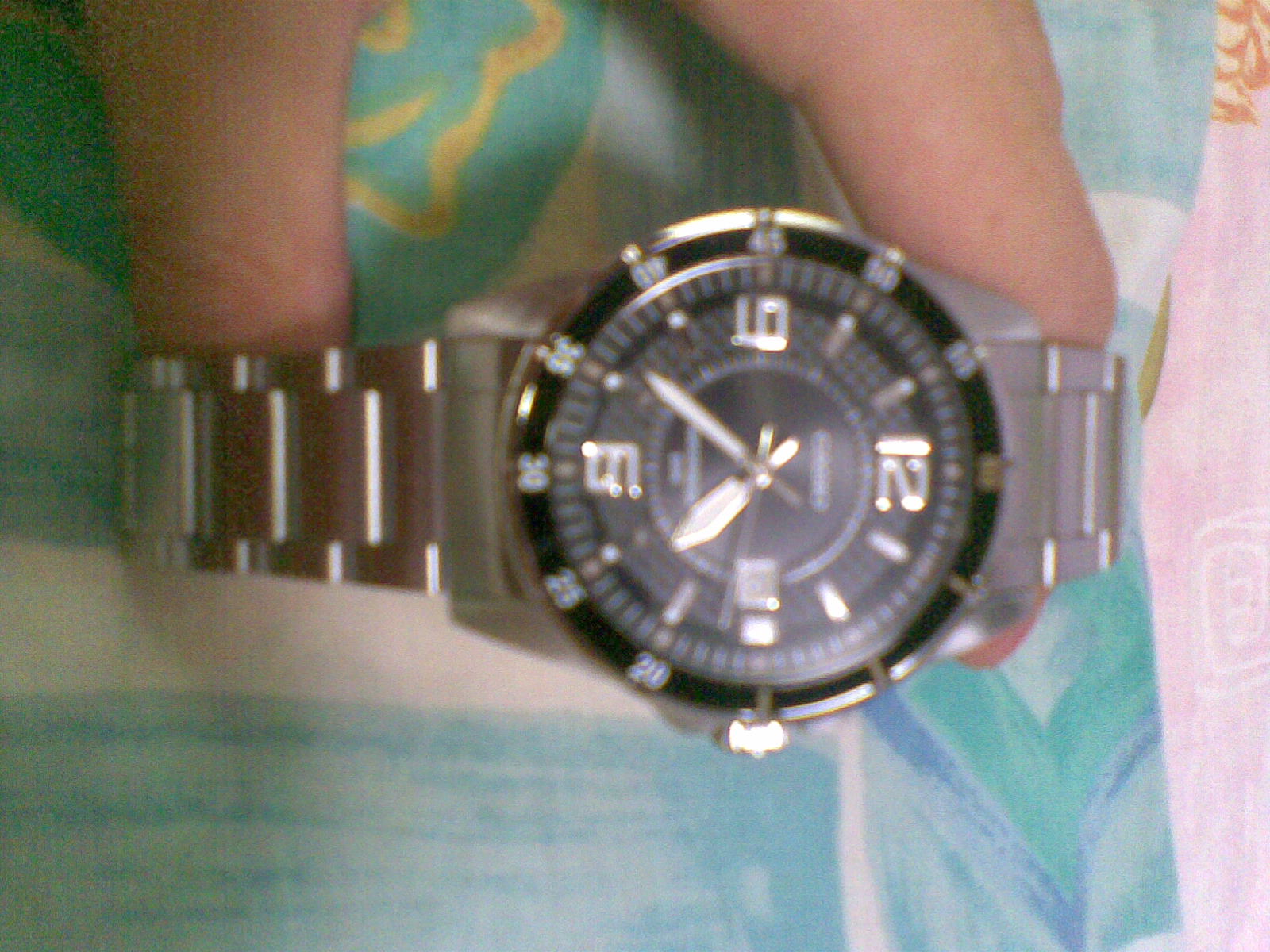A man’s hand extends from the top of the frame, holding a high-quality silver men's watch horizontally between his open thumb and pointer finger. The watch features a band of interlinked metal and a black bezel adorned with numbers at 12, 3, 6, and 9 o'clock positions, while metal dashes indicate the other hours. The face of the watch is meticulously embossed, displaying a combination of gray and white hour and minute hands, along with a prominently long gray second hand. The background consists of a striped pattern in blue-green hues, mimicking the texture and design of a cloth, accentuated with aqua blue, green, yellow, and pink along the right edge, reminiscent of a hospital curtain. The overall scene suggests a juxtaposition between the elegant timepiece and the colorful, patterned backdrop.